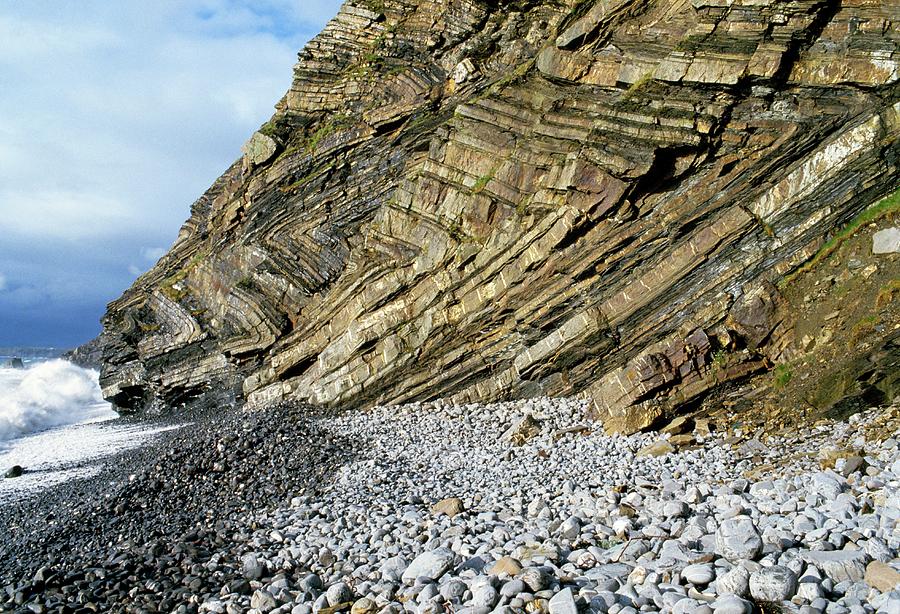This photo captures a striking, striated rock formation meeting the ocean, characterized by its layered, tan and brown hues. The rock, occupying the upper half and right side of the image, displays a complex pattern of ridges and layers that lean at various angles, giving an impression of an aged and weathered surface. The foreground features a band of large, gray pebbles stretching about a third of the way up the photo, reminiscent of a rocky beach sculpted by heavy surf. To the left, there's a glimpse of the ocean with waves crashing against the rock base, and above this, a patch of blue sky filled with hazy white clouds adds a serene contrast to the rugged landscape below.